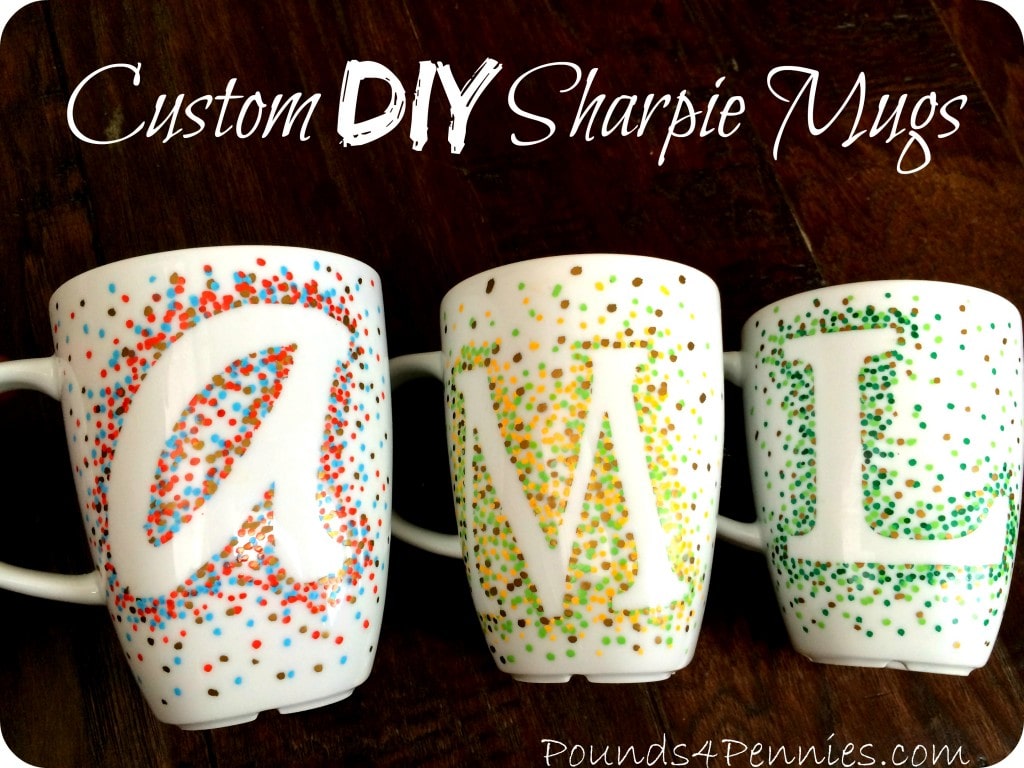This social media graphic features the text "Custom DIY Sharpie Mugs" at the top, written in a sharpie font. Below this text, the graphic showcases three white ceramic mugs laid on their sides atop a dark, wood-grain table. The image is a bird's eye view, highlighting the personalized designs on each mug. 

The mug on the left displays a lowercase cursive "a" surrounded by red and blue polka dots. The middle mug features an uppercase "M" adorned with yellow, brown, and green polka dots. The right mug has an uppercase "L" embellished with brown and various shades of green polka dots. Each mug’s handle is oriented to the left. At the bottom right corner of the image, the web address "poundsforpennies.com" is visible.